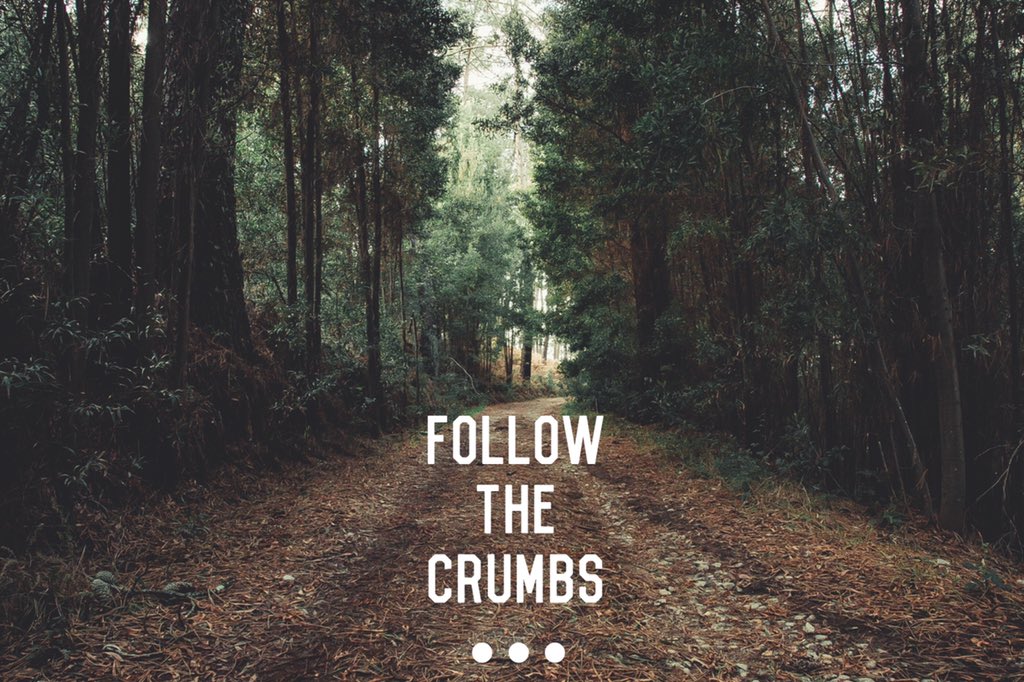This is a detailed color photograph depicting a serene, unpaved trail winding through a dense forest. The path, composed of loose gravel and rocks, is centrally positioned and extends into the distance, slightly curving out of view. The ground is sporadically covered with brown leaves and wood chips, adding to the natural, off-road ambiance. Tall trees with dark green foliage frame the trail on either side, their trunks rising towards the top of the frame and casting shadows that create a muted, almost mystical atmosphere. Light filters through the dense canopy, illuminating parts of the path and highlighting the more vibrant green leaves further down. There are no people or animals present, enhancing the sense of solitude and peacefulness. Near the bottom center of the image, white text reads "follow the crumbs," accompanied by three white dots below it, lending a whimsical touch to the scene.